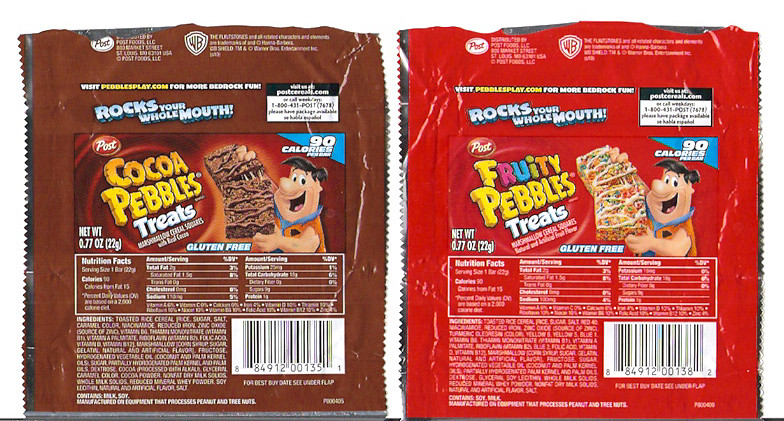The image showcases two packages of Fruity Pebbles cereal treats. On the left, there is a yellow package labeled "Cocoa Pebbles Treats" with a brown background and white text. On the right, there is a red package labeled "Fruity Pebbles Treats" set against a vivid red background, featuring a smiling Fred Flintstone illustration. The overall backdrop of the image is white, highlighting the colorful packaging and appealing appearance of these sweet cereal treats.